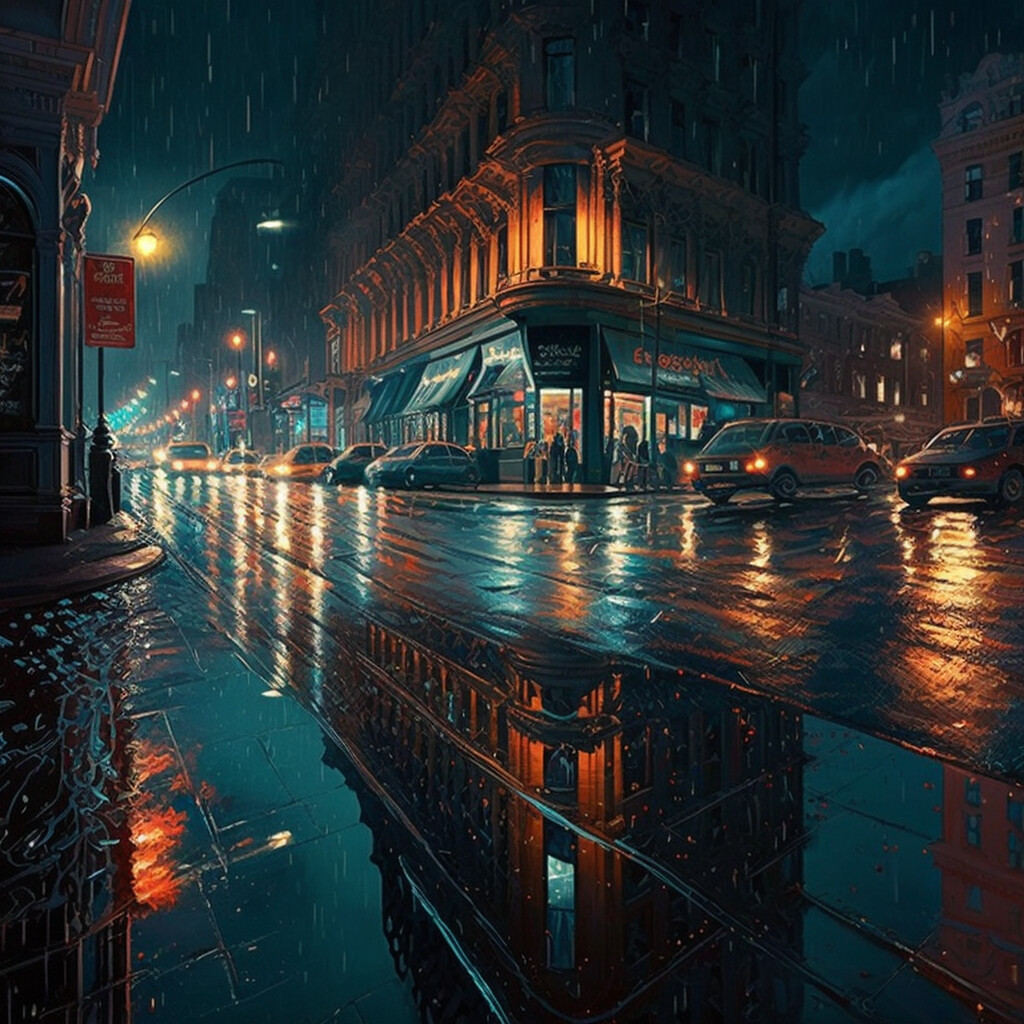The digital illustration captures a rainy night scene at the intersection of a city street, featuring a prominent flat iron building at the corner with an acute angle. The street is bustling with people and activity, illuminated by various lights in medium blue and yellowish-orange hues from street lamps and car headlights. The shiny, rain-soaked road reflects the urban vibrancy, including the tall building and its surrounding storefronts with awnings on their first level. About five cars are parked along the street, with one actively driving on the right side of the image. A red street sign with white text is visible on the left, adding to the scene's authenticity. Rain droplets are distinctly depicted falling in the upper left, and some clouds are visible in the upper right, enhancing the atmospheric depth.